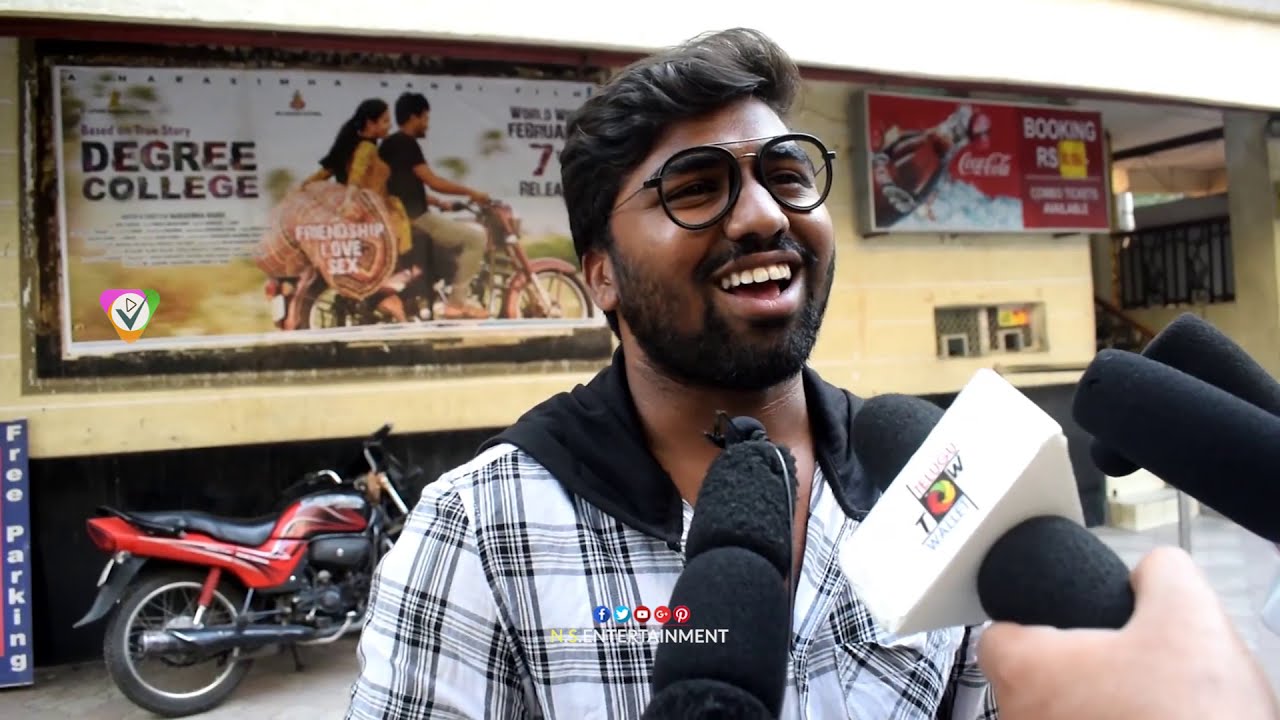A dark-skinned man, seemingly of Indian descent, is being interviewed by multiple news sources. His hair, approximately three to four inches long, is dark and slightly curls around his head. He wears black-rimmed glasses and is smiling broadly, revealing his top row of teeth. The man dons a predominantly white jacket with black stripes forming small squares and a solid black hood.

In front of the man, four black microphones are positioned closely; one has a white box indicating its news company. Logos for Facebook, Twitter, YouTube, Google+, and Pinterest are visible next to the text, "something entertainment," on a strip in front of him.

The background features a red motorcycle parked to his left and a yellow wall adorned with advertisements. On the man’s left is a billboard advertising a college degree with an image of a guy and a girl riding bicycles. On his right, towards the top of the wall, there's a Coca-Cola advertisement. The setting appears to be either an outdoor street or a brightly lit indoor space resembling a hotel entrance.